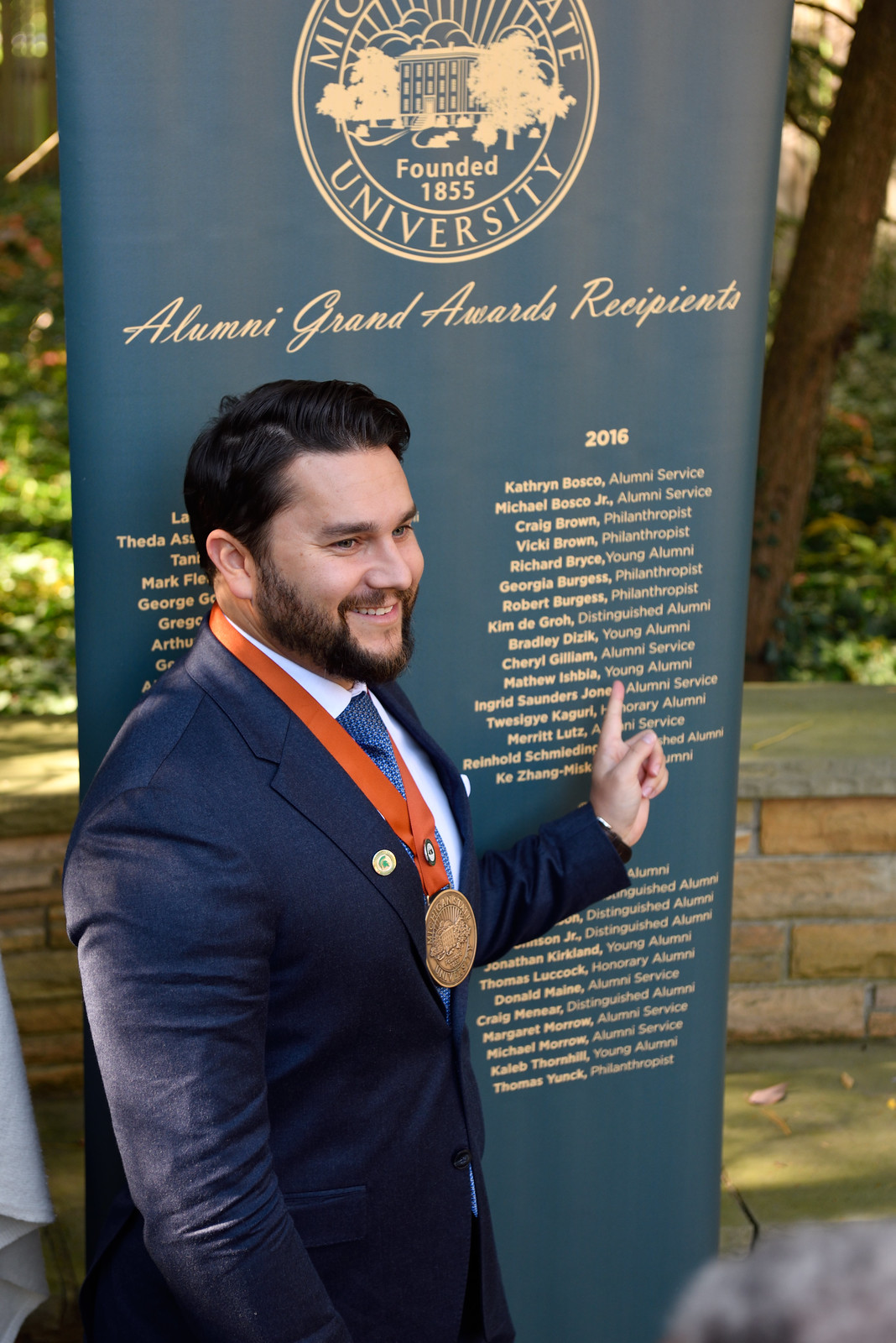This color photograph captures a young man standing outdoors in front of a dark green banner with gold writing, partially obscured but identified as associated with Michigan State University, founded in 1855. The banner reads "Alumni Grand Awards Recipients" and lists multiple years with corresponding names. The young man, who is tall and fair-skinned with a medium complexion, has dark brown to black hair and sports a beard and mustache. He is dressed in a navy blue suit with a white shirt and a dark blue tie adorned with white dots. A gold lapel pin decorates his right lapel.

Around his neck hangs a large circular medal on an orange ribbon. With a smile and an expression of looking off into the distance, he points with his left hand to the year 2016 on the banner, specifically highlighting the name "Matthew Ibbani Ishbia" under the "Young Alumni" category. The background features a sunny afternoon scene with trees and a low brick bench, indicating that the photo was taken outside.